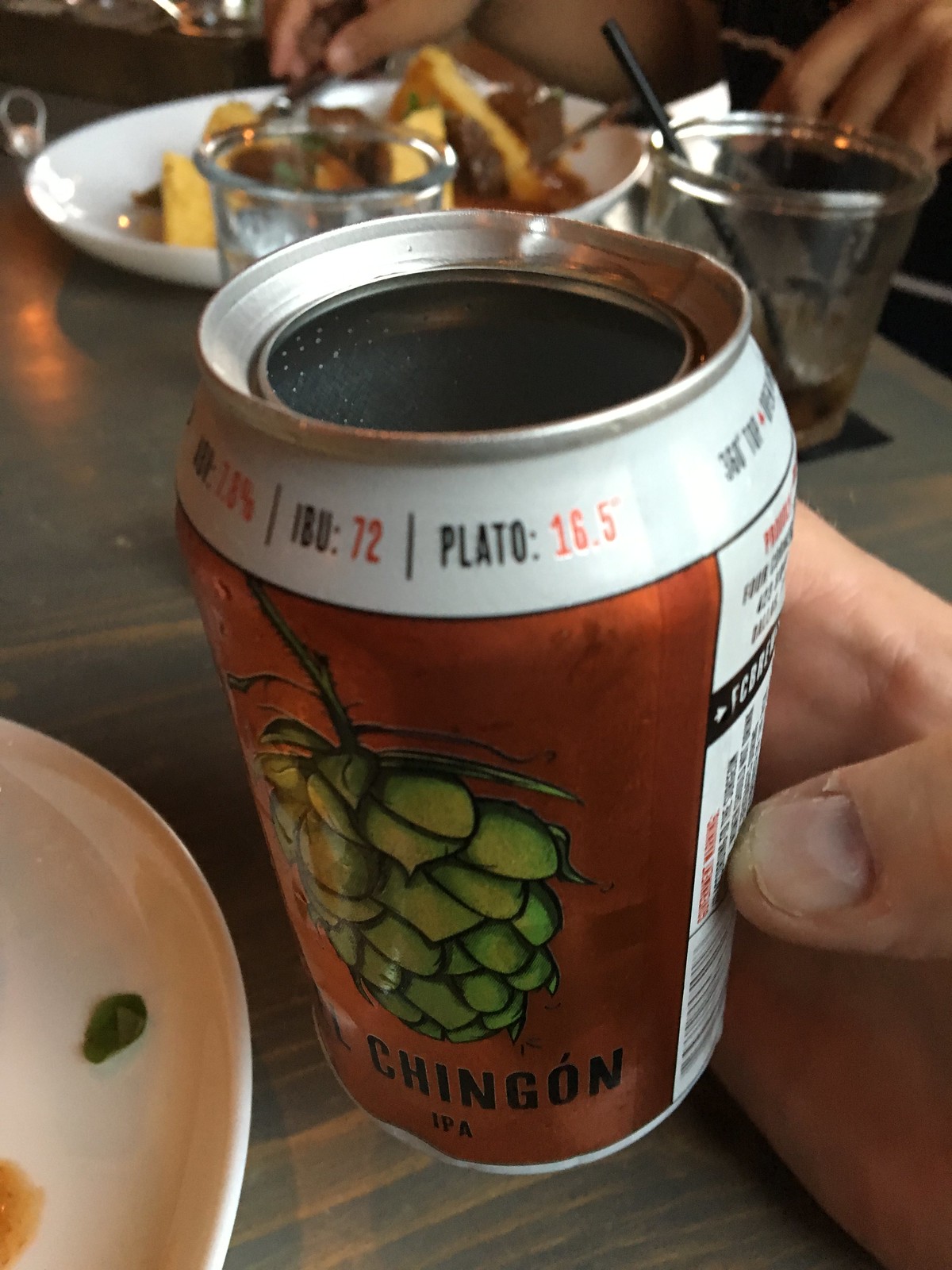The image captures a close-up view of a scene where people are dining. Dominating the foreground is a brown wooden table with lighter brown stripes adding texture to its surface. On the left-hand side, partially visible, is a white round plate with a green item and a smear of red sauce. Adjacent to this plate, a person's right hand, with fair skin, holds a beverage can labeled "PLATO" in bold black letters, "16.5" in red, and "IBU 72" in black, bearing an image of green grapes and the text "CHINGONIPA" in black. In front of this person, two cups are present; although one is mostly obscured by the can, the other is more visible, featuring a black straw and filled with a brown liquid, resting atop a black napkin. The intricate details hint at an intimate dining experience amidst conversation and shared meals.